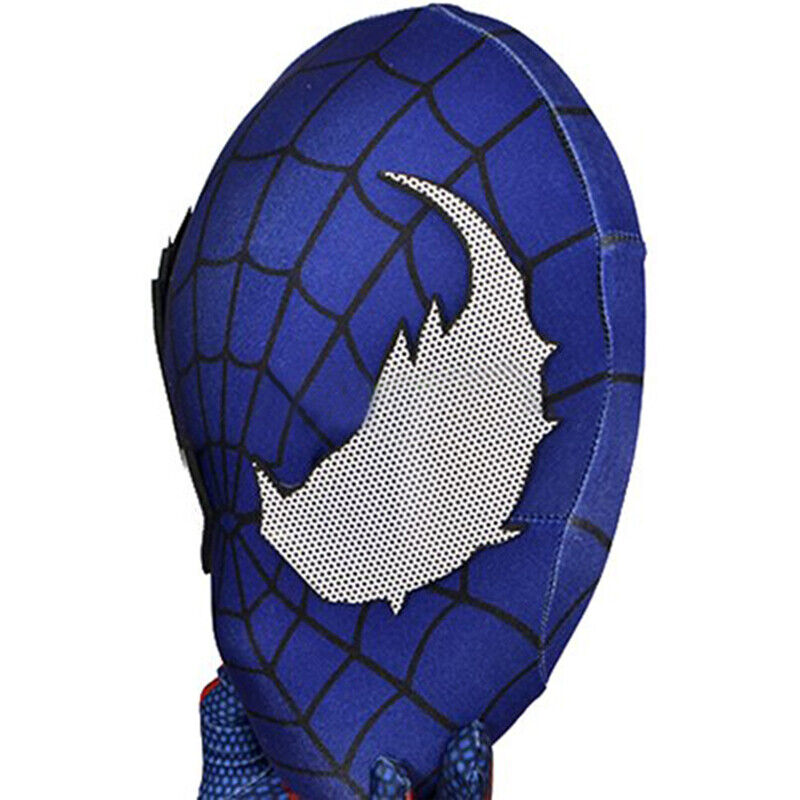The image is a full-color, vertically rectangular photograph of a blue Spider-Man mask. The mask features a prominent, large right eye with a white mesh and small holes, allowing visibility for the wearer. The design on the mask includes the classic black web pattern, but in this variation, the mask is entirely blue. The aesthetic detail of the eye closely resembles that of Spider-Man’s villain, Venom, emphasizing an elongated, elliptical shape. The mask is being held by a gloved hand, with three fingers visible in the lower left-hand corner. The glove is part of the costume, matching the blue hue of the mask but decorated with light blue or white dots. The image focuses solely on the front of the mask, showcasing the forehead, nose, and right eye, with no additional background elements visible.